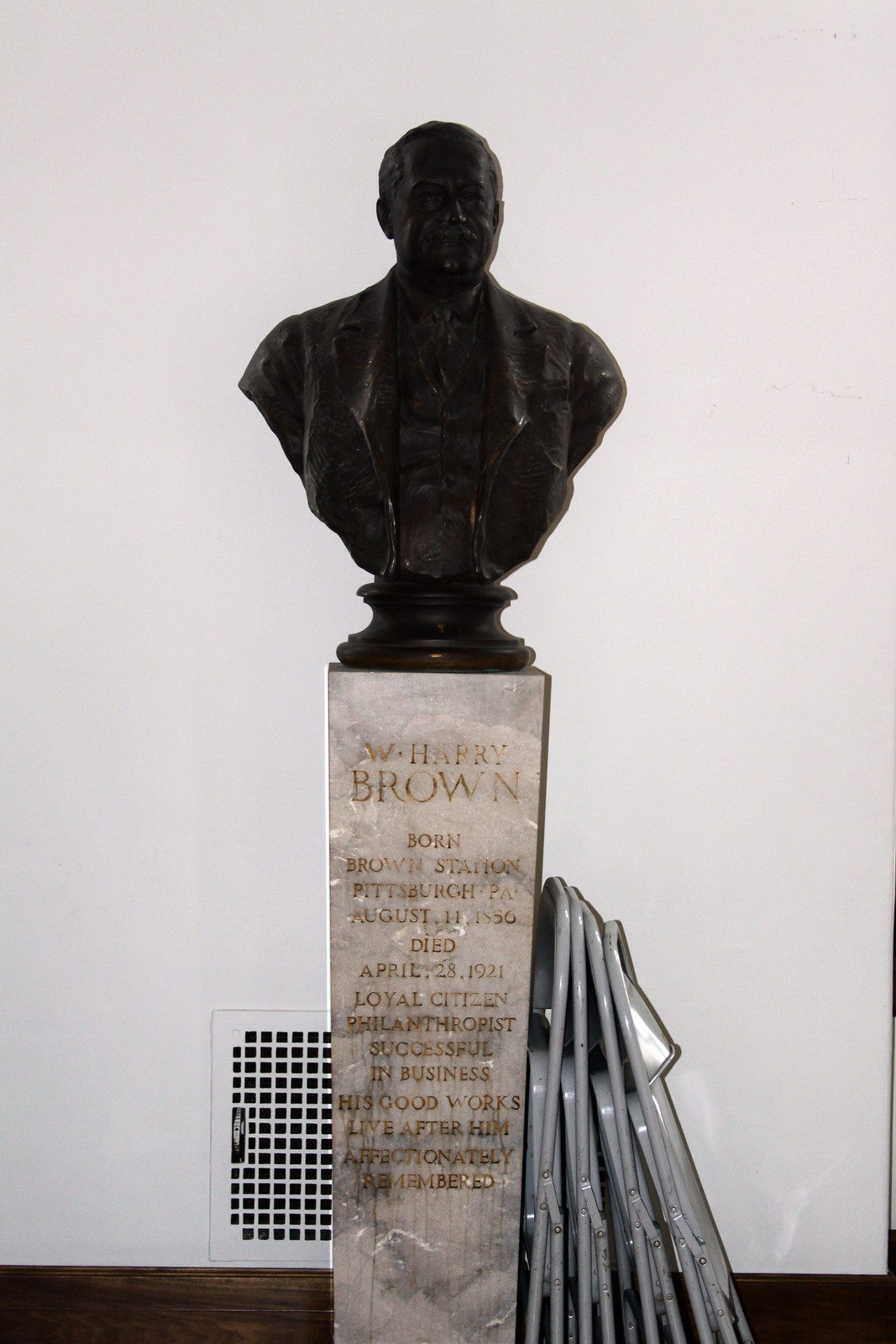The photograph showcases a dark bronze bust of a distinguished-looking man with receding hair and a bushy mustache, perched on a marble pillar. The man has a square jaw accentuated by rounded cheeks and is dressed in an old-timey suit with a tie, though specific details of his clothing are obscured due to inadequate lighting. The marble pillar bears an inscription that reads: "W. Harry Brown, born Brown Station, Pittsburgh, Pennsylvania, August 11th, 1856 - Died April 28th, 1921, loyal citizen, philanthropist, successful in business, his good works live after him, affectionately remembered." The scene also includes four folding metal chairs leaned against the right side of the pillar and a heating vent on the wall behind it.